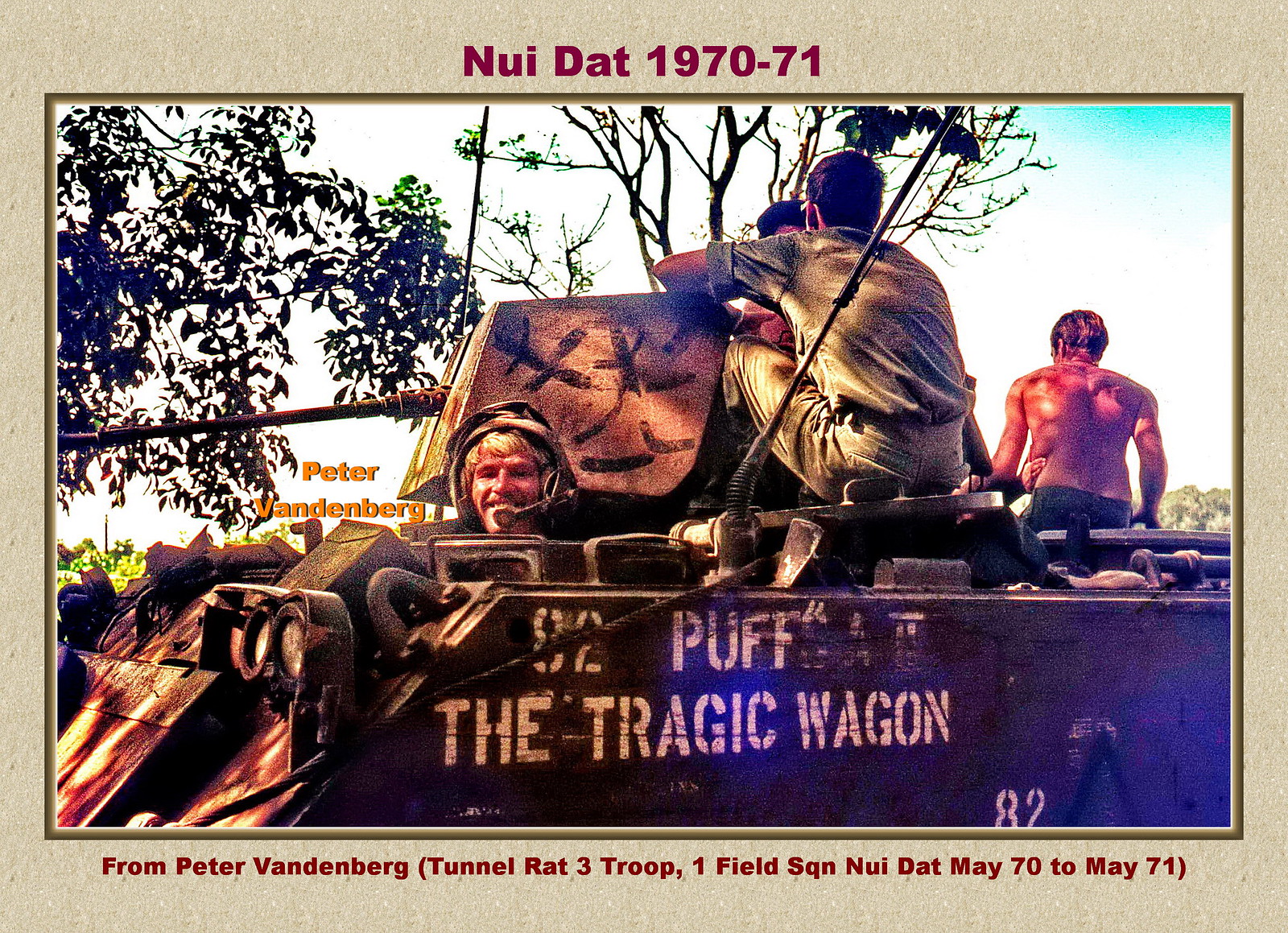The image features a tan matte border surrounding a rectangular photograph, emblazoned with the inscriptions "Neu Dat, 1970-71" on the top in a purplish hue and "From Peter Vandenberg, Tunnel Rat 3, Troop 1 Field, SQN Neu Dat, May 70-May 71" in red at the bottom. The central focus of the image is a military tank prominently positioned in the center, distinctly labeled on its side in white letters as "82 Puff the Tragic Wagon". A man, identified as Peter Vandenberg by adjacent text, emerges from the front of the tank, wearing a headset. The tank carries several soldiers on top. The scene is set outdoors, likely in Vietnam, with a backdrop of trees and a sliver of sky visible at the top. The image is vibrant with colors including tan, purple, brown, green, red, and yellow, indicating a daytime setting during the years 1970-71.